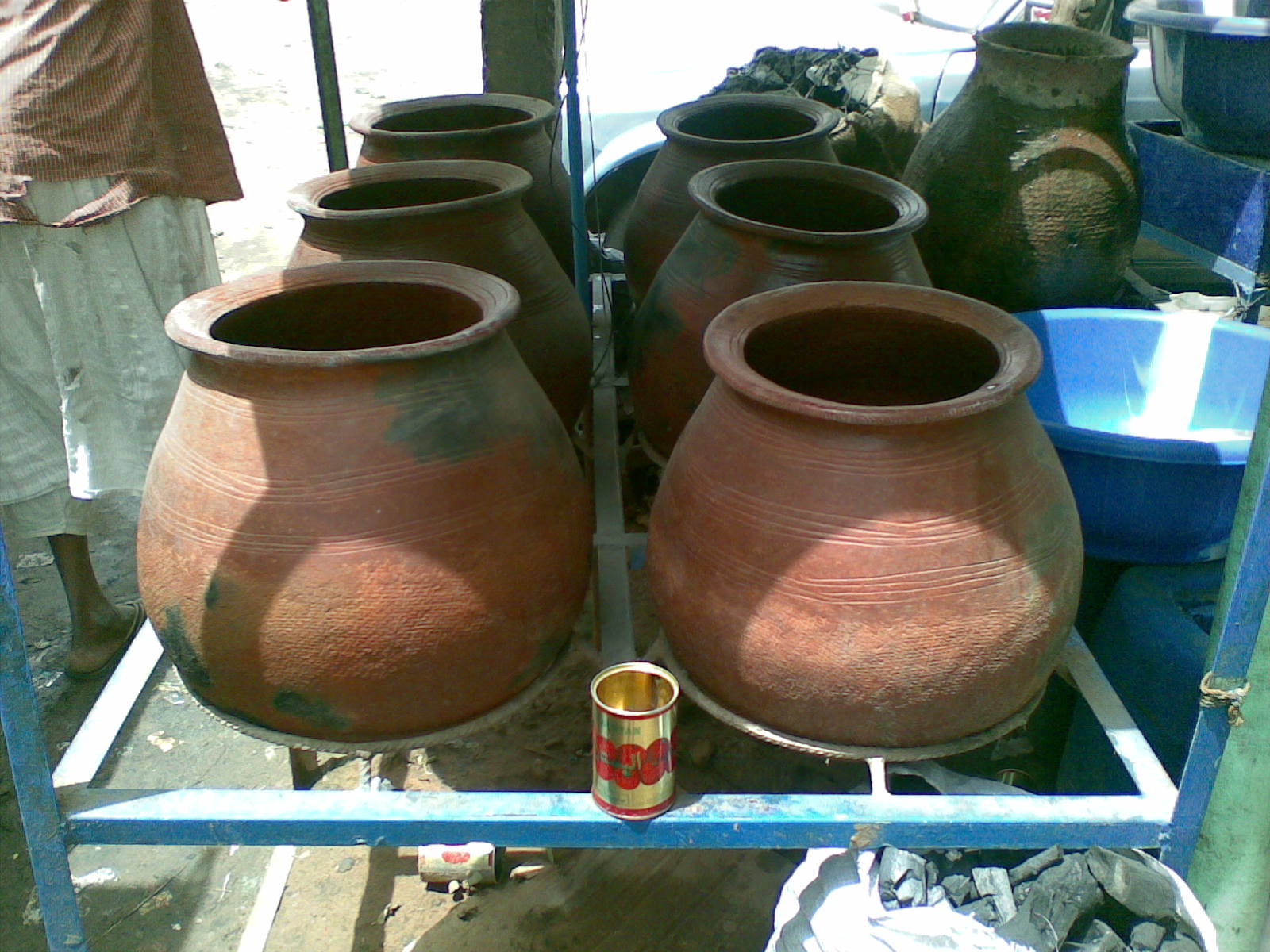In this outdoor photograph, likely taken during the daytime given the bright, washed-out background, a blue metal rack stands prominently in the shaded foreground. The rack holds rows of six large clay vases or urns, each resting securely on metal rings. The vases are arranged in two rows of three. Positioned in the front center of the rack is a cylindrical, golden-colored can adorned with red logoing. 

On the left edge of the image, partially cut off, is a person wearing a torn, perhaps brown or striped shirt, and white shorts or a white skirt, along with sandals. To the right of the blue rack sits a large blue basin, possibly with something white being poured into it, and another sizeable dark brown vase. At the bottom of the frame, a bag containing what appears to be black charcoal or rocks is visible, contributing to a sense of an open-air market setting.